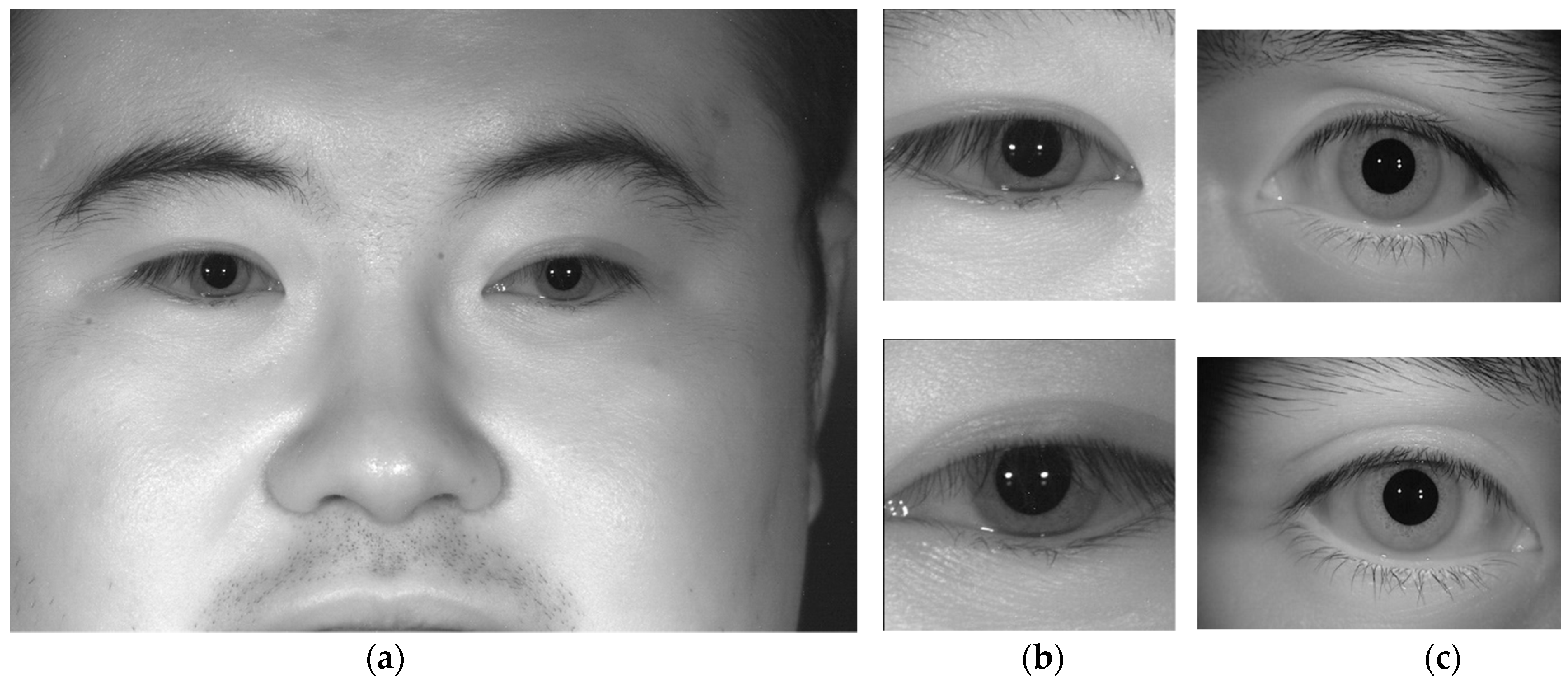The image is a composite featuring five distinct pictures, with the largest on the left and four smaller ones aligned to its right. The primary photo to the left is a close-up, black and white image capturing the face of an Asian man from his forehead down to his upper lip. The man, whose face appears chubby, has small, dark eyes with black eyebrows, a flat nose, and a faint beard above his lip. The focus and apparent use of night vision give his eyes an almost innocent expression.

To the right, the four smaller images each emphasize an eye. The top two images feature eyes with dark irises surrounded by slightly darker rims, hinting at a uniform eye color. In contrast, the bottom two eyes have much paler surroundings, though their irises remain black. These various eyes exhibit different emotions and postures, suggesting a study on the range of expressions and movements eyes can display, creating a dynamic contrast to the prominent, stoic face on the left.